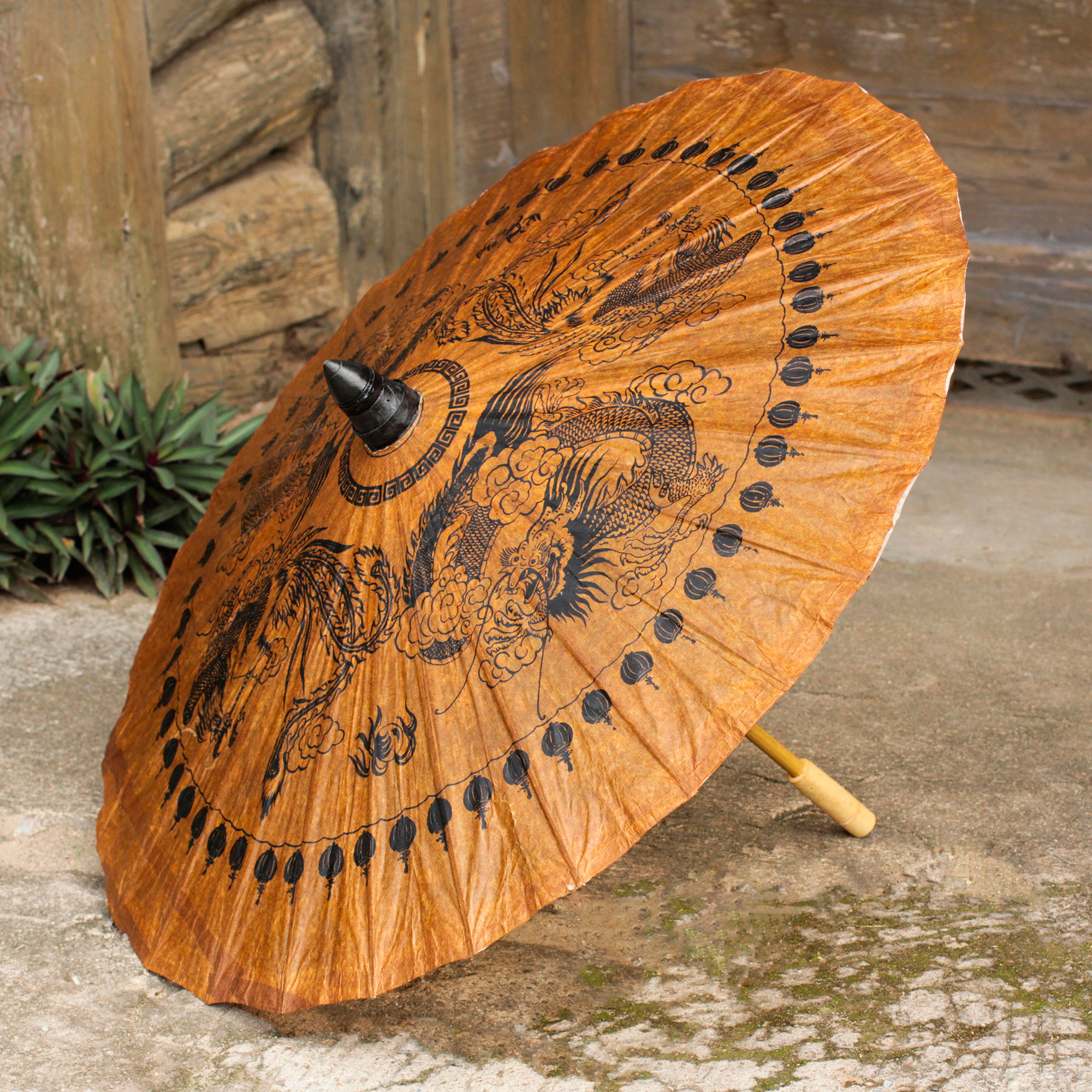This is a four-color, vertically rectangular photograph, seemingly taken outdoors in natural daylight after a rain. The main focus is an open, orange umbrella with intricate, black artistic designs depicting several Asian-style dragons amidst swirling smoke, accented by a black circular border near its edge. The top of the umbrella features a prominent black point, and it rests on a light gray hard surface, possibly concrete or stone, with a handle that is short, wooden, and brown, extending out to the right with a thicker, lighter-colored piece at the bottom. The umbrella appears to be made of thin, potentially flimsy material resembling taffeta paper.

In the background, primarily on the left side, there is a small green plant visible, contrasting with the wood elements behind it. The top portion of the background is dominated by walls resembling log cabin construction, with wood extending towards and off the right edge of the image. The ground in the lower right corner of the image appears to be wet, though it could also be moss. Overall, the scene evokes a post-rain setting, with the umbrella laid out, possibly in disuse or abandonment.